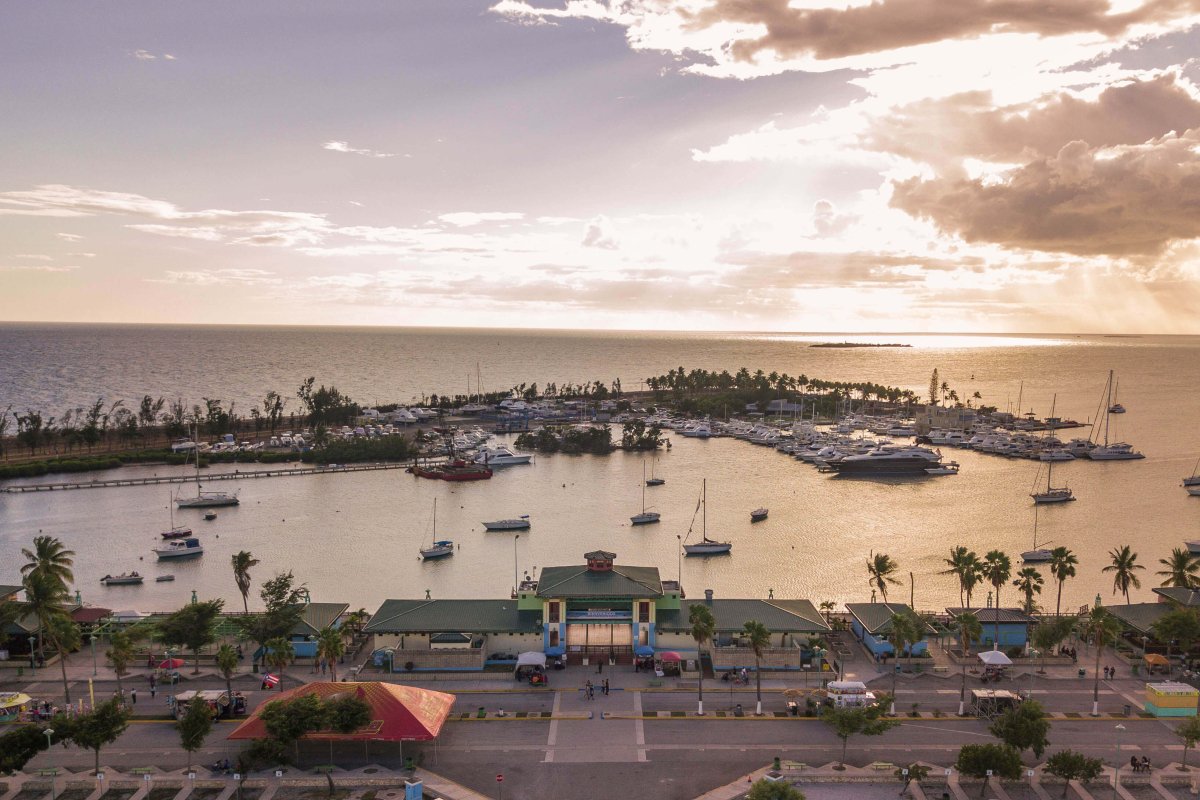This photograph captures a serene harbor scene at sunset in a coastal resort town. In the foreground, a street lined with rows of palm trees frames a terminal building with beige stucco walls and green roofs, featuring a central tower with a blue base, beige top, and a red circular design. Few people are seen walking on the street. Behind the terminal, a rectangular marina teems with small, white sailboats with their sails down. Adjacent to this marina, a pier extends diagonally to the right, lined with green trees and filled with various watercraft, including a large yacht at the end of the left-hand pier. The harbor is bordered by the calm ocean waters, transitioning from blue to golden hues with the setting sun. In the distance, a small dark island sits against a backdrop of golden-lit water. The sky above is a pale blue, clear on the left with scattered clouds on the right, some tinged with light brown or gold, and a burst of white where the sun is, casting rays that illuminate the scene with pinkish and blue tones.